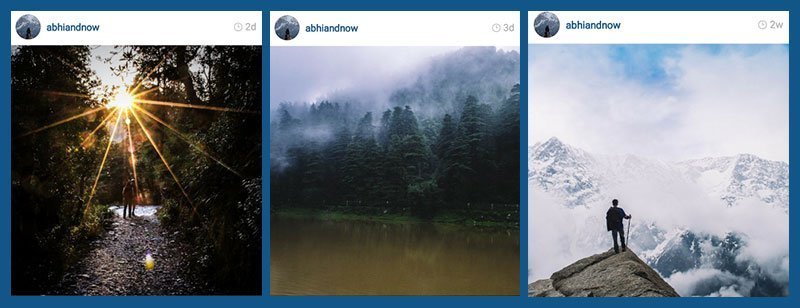This image is a screenshot from an unspecified website, showcasing three square photos arranged horizontally. Each photo is separated by a thin blue border and topped with a white banner. In the white banner above each image, there is a small, round profile picture with a blue background, likely depicting a landscape. The user's name, "ABHIANDNOW," is displayed next to each profile photo.

From left to right:

1. The first photo captures a stunning forest scene. Sunlight filters through the dense trees, casting beautiful sun rays that illuminate the forest floor and create an enchanting atmosphere.
   
2. The second photo features a landscape where fog-covered mountains loom in the distance. Closer to the viewer, pine trees populate the scene, and at the bottom of the photo, a murky, brownish lake adds an element of rugged natural beauty.

3. The third photo highlights a breathtaking vista of snow-capped mountains. At the lower left of the image, a cliff juts out, with a solitary silhouette standing at its edge, gazing into the expansive mountainous horizon.

The combination of these three distinct landscapes provides a visually captivating and serene representation of nature's diverse beauty.